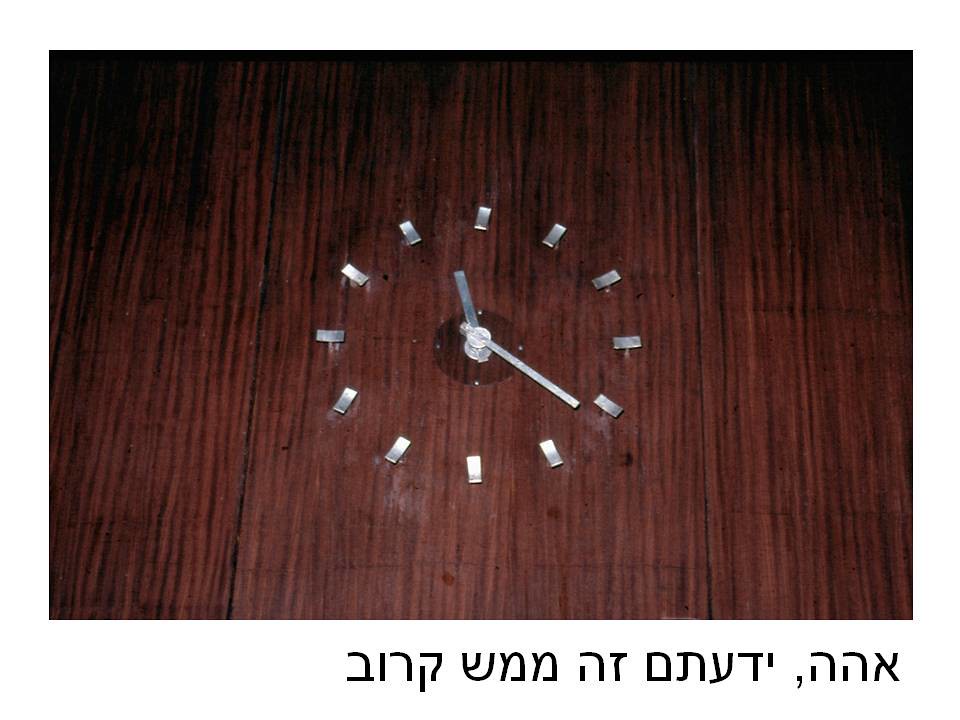This detailed photo captures a close-up of an unconventional wooden clock face, distinguished by its dark brown wood adorned with subtle black creases. The clock features minimalist design elements, with twelve small silver metallic strips marking the hours in place of traditional numbers. At the center of the clock is a clear circle, onto which two slender silver clock hands are affixed—the minute hand being notably longer than the hour hand. The time on the clock appears to be set around 11:22 or 11:23, likely PM, given the dark ambiance of the photo, which seems illuminated by a flash. Below the clock, against a white background, there are inscriptions in a foreign language, although the specific language is indiscernible to the viewer.